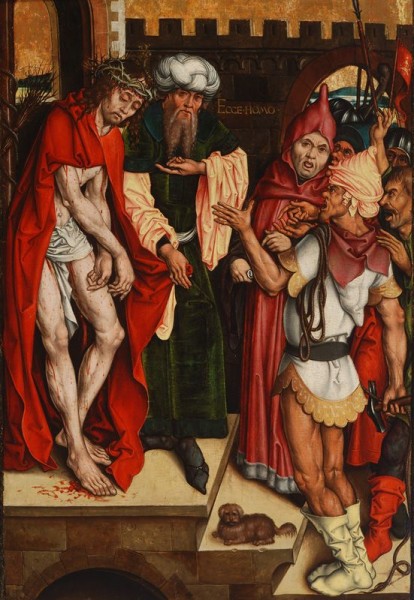This detailed painting, likely from the Renaissance era, depicts a poignant religious scene featuring a nearly naked, bloodied Jesus with a crown of green thorns, standing on a podium. Around him, several figures are portrayed with intense expressions and dramatic gestures. To his immediate right, a man in an elaborate white turban and green robes with yellow sleeves points towards Jesus. Directly behind this man, another figure in a red gown with a pointed hood stands with an open mouth, seeming shocked or distressed.

On the left side of the panel, stepping down from the stone podium, stands a man in a green cloak, aligning with an observer in tall white boots and a white tunic adorned with gold trim. The latter holds a hammer, perhaps a Roman soldier, indicating the aftermath or preparation for the crucifixion. Surrounding them on descending steps, a group of men in various medieval or Roman attire, some in white and gold dresses, show an array of emotions from anger to astonishment. The background reveals castle ramparts, and there is a segment of writing centrally placed within the artwork, further emphasizing its historical and narrative depth. The composition and attire of the figures, alongside the architectural elements, underline the scene's historical and cultural significance.